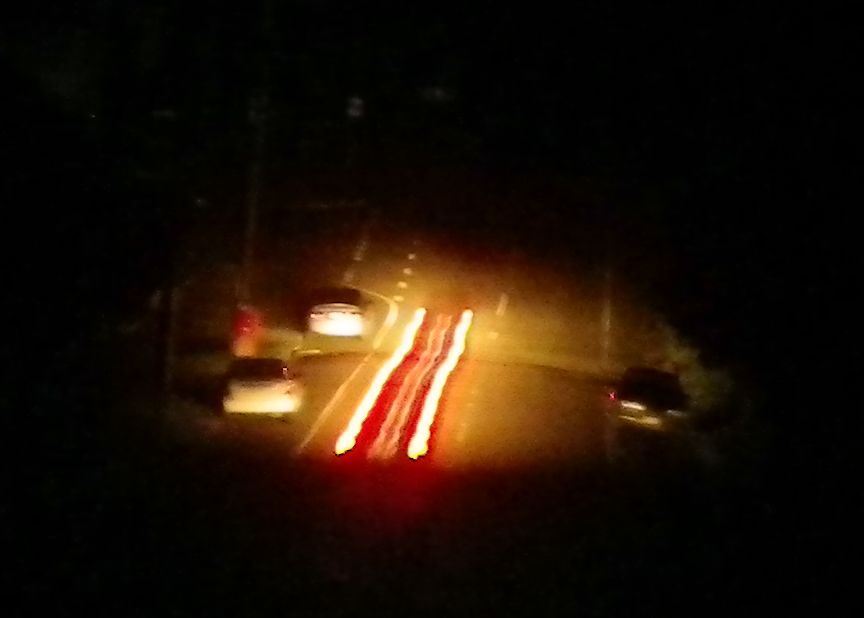The photograph is a color image captured at night, featuring a dark background with a central illuminated, slightly flattened oval shape. The scene reveals a highway with distinct, blurred lines and several elements suggestive of motion and light effects. On the right side, the front lights of a truck heading in the opposite direction shine through the darkness. An empty lane lies next to it. To the left of this lane, a striking visual effect shows orange and red streaks, resembling tire marks on fire, extending horizontally across the road. Further left, two white cars are visible, traveling in the opposite direction. A small red object is positioned to the left of the car closer to the camera, adding a point of intrigue in the composition. The highway markings, including a muted white line and various broken lines, are illuminated within the oval light. The overall image is blurred and dark, creating an abstract and somewhat ethereal night scene filled with a golden, almost rope-like light effect in the middle of the street.